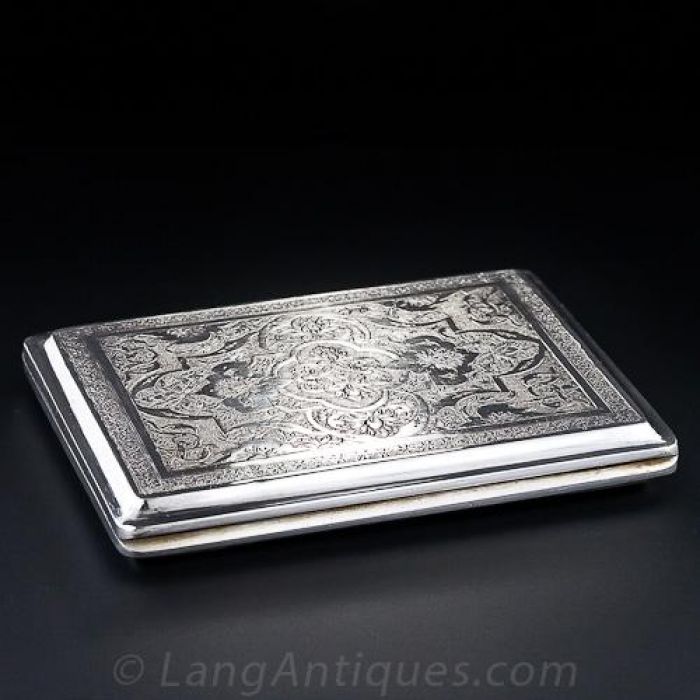The image presents an overhead and slightly angled view of a rectangular, silver container with intricate engravings. The background transitions from black at the top to various shades of gray, lightening towards the bottom. The container, which appears flat and slim, is crafted from silver and features detailed etchings, including floral designs and patterns. The top of the container is just slightly ajar, revealing that it is a case with both a top and bottom part. Light reflections enhance its shiny, metallic surface. In light gray text across the bottom, it reads "LangAntiques.com". The overall composition suggests a meticulously designed and polished item, possibly a decorative or collectible piece.